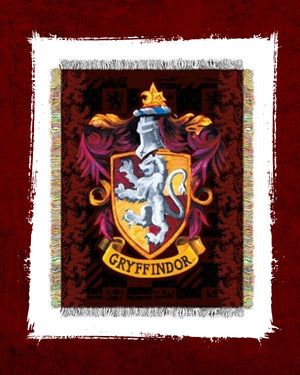The image shows a detailed portrayal of the Gryffindor house crest from the Harry Potter series. The outermost border is a deep maroon or red square, encapsulating a white-framed section with rough, frayed edges. Inside this white frame lies another maroon-colored interior border. The centerpiece is the Gryffindor shield, displaying bold colors of yellow and red, divided diagonally. Adorning the crest is a prominent lion in a reddish stone-gray hue, standing on its hind legs with its claws outstretched and its tail flopping downward. Purple and magenta feather-like designs embellish the top and bottom of the shield. A knight's helmet sits atop the crest, adding to its regal appearance. Beneath the shield, a yellow ribbon is inscribed with "Gryffindor," tying together the majestic and spirited theme of the image.